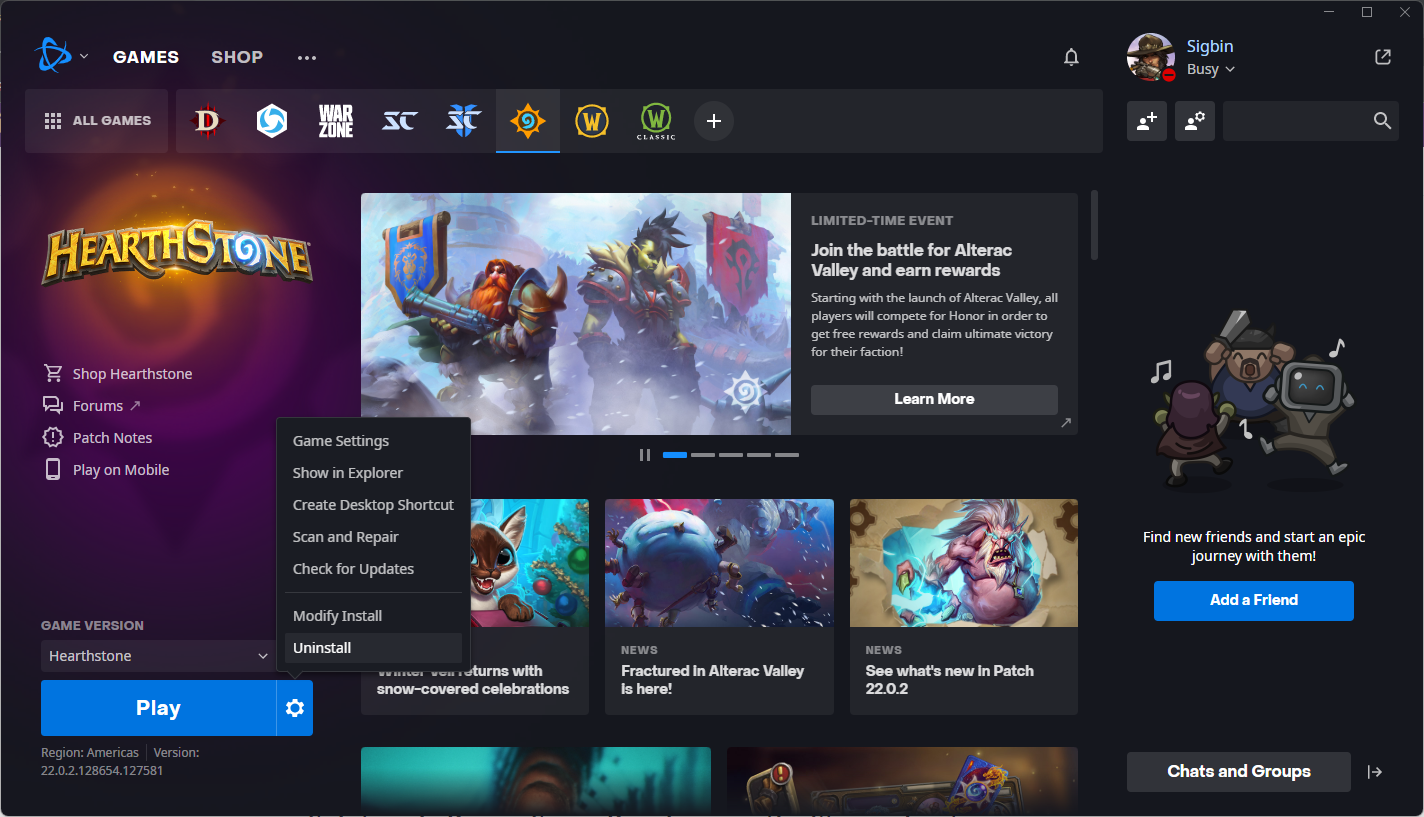This image is a cropped screenshot of the desktop version of Battle.net, a popular gaming platform. The background is predominantly black. 

At the top left corner, the Battle.net logo is prominently displayed, featuring a design of blue interlocking planets. To the right of the logo, the navigation options "Games" and "Shop" are shown in small, bold grey letters, with "Games" being highlighted in white to indicate its selection.

Directly below these options is a dropdown box labeled "All Games." A long rectangular bar adjacent to this box displays various game logos, representing the games available in the user’s Battle.net account. These include titles like "Call of Duty: Warzone," "World of Warcraft" and its expansions, as well as "Hearthstone." 

"Hearthstone" is currently selected, which brings up a detailed interface related to the game. Towards the bottom left of the screen, a prominent blue "Play" button is positioned, above which the "Hearthstone" logo is displayed at the top left of this section. In the middle section, there are several options such as "Shop Hearthstone," "Forums," "Patch Notes," and "Play on Mobile."

To the right of these options, the game’s information panel provides updates like limited-time events and recent news, highlighted by a notification about the latest updates in patch 22.2.

On the top right, a vertical panel contains the user’s profile information, featuring the username and a user profile picture on the left. Below the username, a friends list is visible, completing the social aspects of the Battle.net interface.